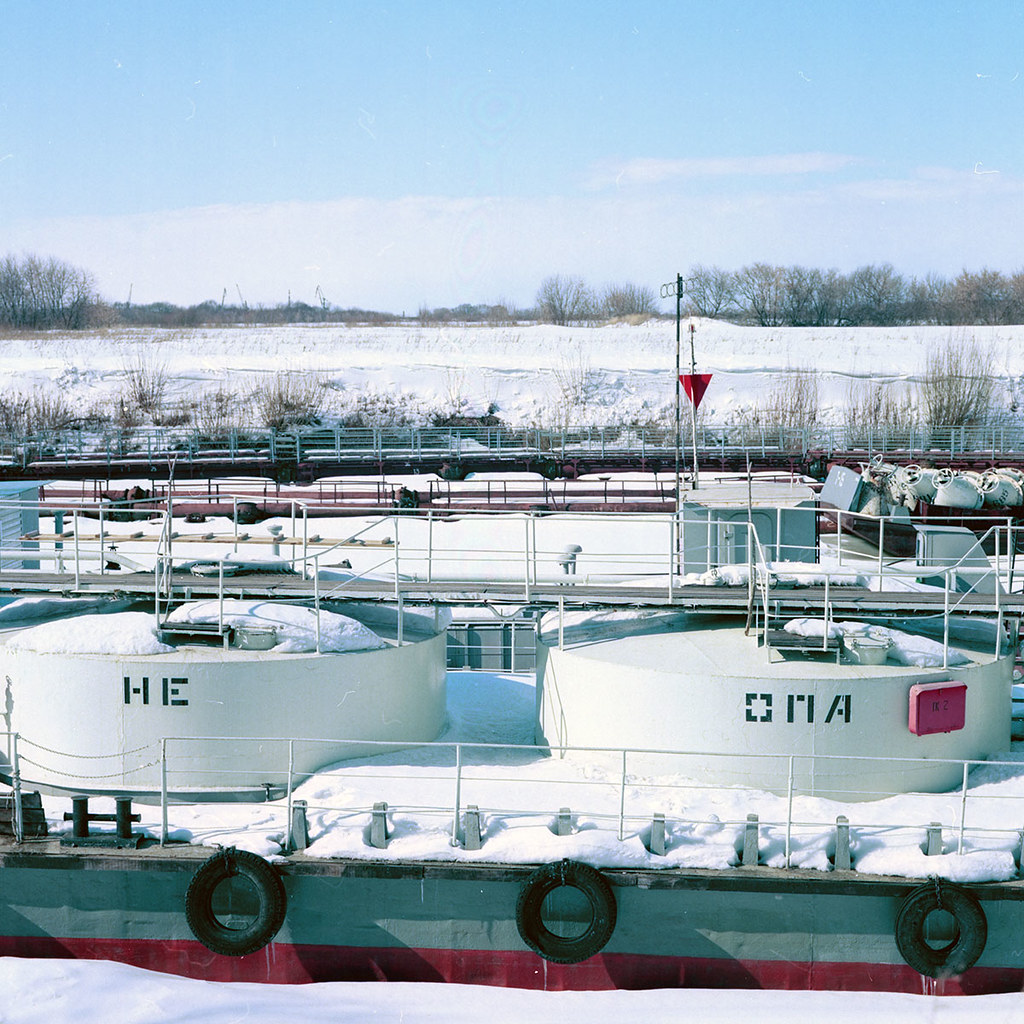The image depicts a snowy commercial dock area with a portion of a ship in the foreground. The sky above is a pale blue with thin white clouds near the horizon, which meets a snowy landscape dotted with sparse shrubs and trees in hibernation. The scene is dominated by a mix of bright and subdued colors, including large stretches of white snow, a green stripe, and a red stripe on the ship, along with sprinkles of blue and gray that give the scene a wintery feel. Prominently mounted on the ship's side are three tires, providing a buffer at the docking point. Two large cylindrical tanks are situated on the vessel. The left tank is marked with the letters "H-E" while the right one has "O-N-A," though it's unclear if these are English letters or symbols from another language. The ship and dock are potentially bustling with industrial activity, but the snowfall blankets the scene, creating a serene and somewhat desolate atmosphere.